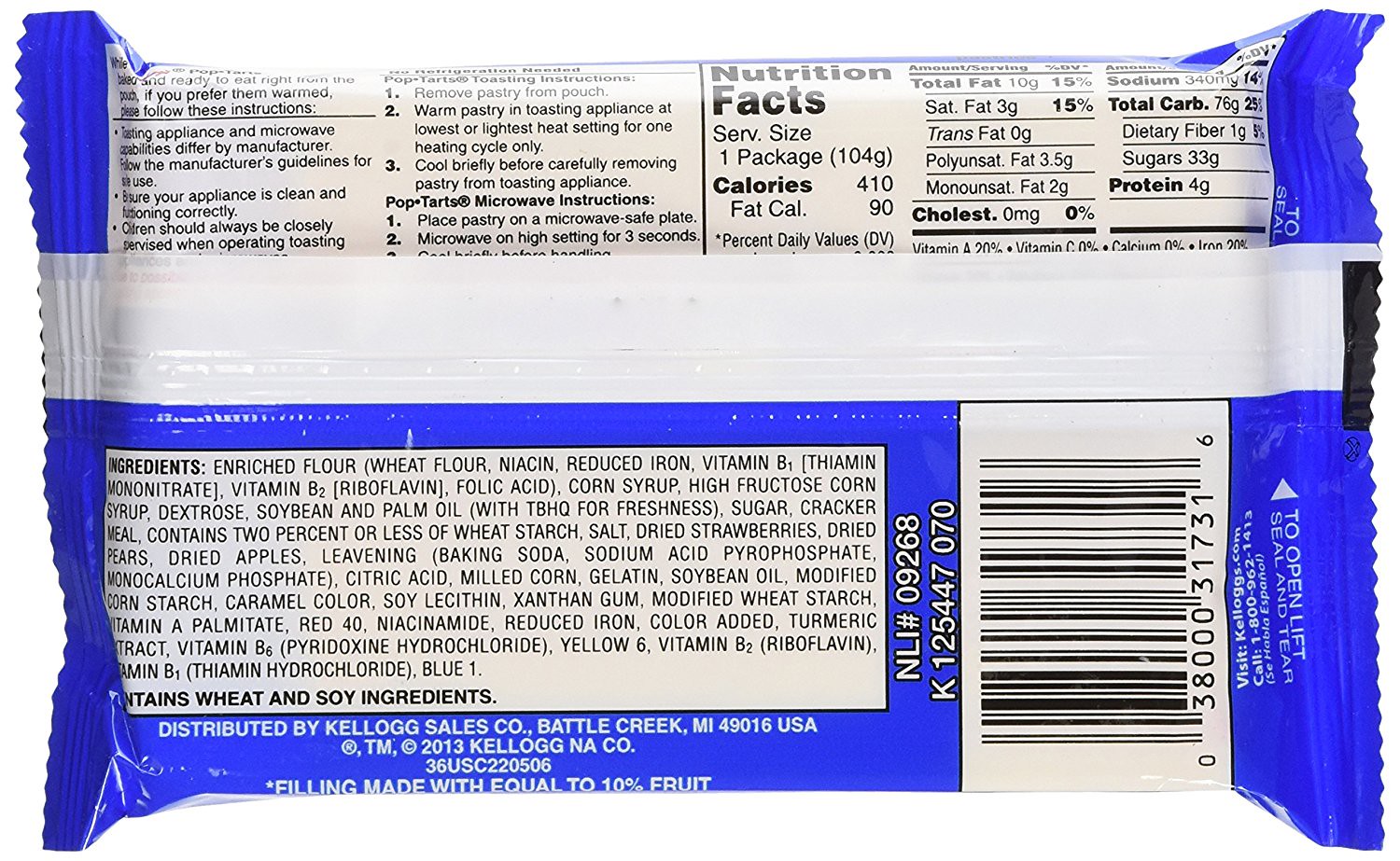This image depicts the back of a blue and white food package, likely a Pop-Tart, distributed by Kellogg's in Battle Creek, Michigan. The overall design is rather plain, with a barcode on the right side and several ridges along the edges. The background of the image is white. The text on the package, written in black, occupies most of the space, including nutritional information in the middle detailing 410 calories, saturated fats, trans fats, cholesterol, and more. The ingredient list on the bottom left mentions enriched flour, wheat flour, niacin, and reduced iron, while further details indicate it contains wheat and soy ingredients. The package also includes heating instructions: to microwave the Pop-Tarts, place them on a plate and heat on high for three seconds. Additionally, each package contains two Pop-Tarts with the filling amounting to 10% fruit.